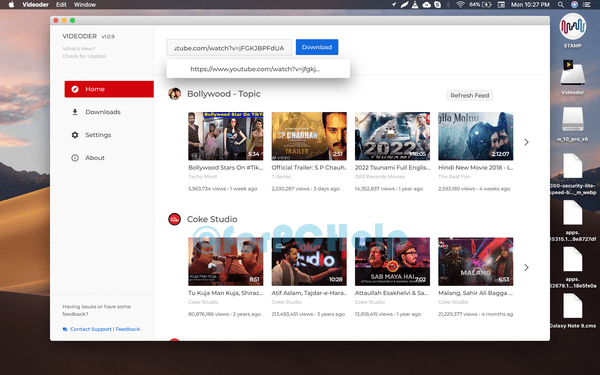The image showcases a MacBook or Mac desktop screen with the familiar Apple user interface. At the top left corner of the screen, the iconic Apple logo is displayed, followed by the text "Video Finder" in bold white lettering. Next to it, in non-bold white text, are the options "Edit" and "Window."

A window is open in the top left corner of the screen, featuring the traditional Mac window controls: a red circle to close, a yellow circle to minimize, and a green circle to maximize or restore the window. Within this window, a menu bar on the left side shows various options in uppercase gray letters. The highlighted text reads "VIDEODER," and next to it, the application version "10.9" is displayed. Below this, there is a smaller, lighter gray text that says "What's New," followed by "Check for Updates."

The primary menu options include "Home," "Download," "Settings," and "About." The "Home" option is currently selected, indicated by a surrounding red rectangle. Below these options, there's a search query bar designed for pasting YouTube video URLs, with a URL already entered. The entered URL appears just beneath the search bar. 

To the right of the search bar is a rectangular blue icon labeled "Download" in white text. Underneath the search bar, there is a user icon featuring two or three faces, which is labeled "Bollywood-topic" in gray text. This section also includes four different icons suggesting varied content categories: the first depicting a fashion show, the second resembling a movie, the third marked with "2022" and showing a patriotic scene, and the fourth indicating a romance-themed category.